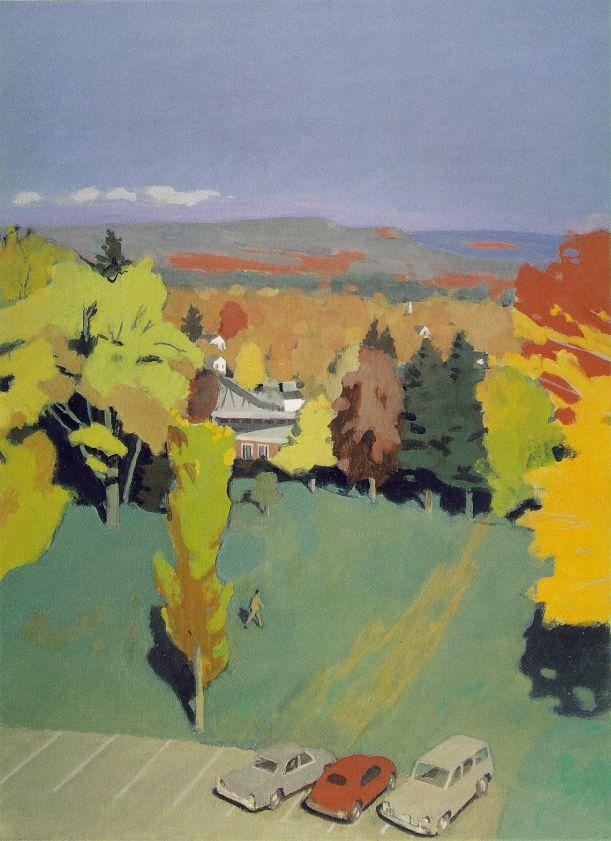This painting captures a serene autumnal scene in a small village set within a forest. At the bottom, a gray parking lot is defined by white lines marking spaces where three vintage cars from the 60s or 70s are parked: a gray sedan on the left, a red rounded-roof car in the middle, and a light brown wagon with open clear windows on the right. Nearby, a person dressed in beige walks across a patch of green grass with a streak of yellow running through it. A single tree with a light brown trunk and a mix of green and yellow leaves stands in this grassy area.

In the midground, there's a building with a pink-colored brick front, two windows, and a slanted roof painted in mostly white and gray hues. This structure appears to be a house or perhaps a church, surrounded by tall trees displaying vibrant autumn colors—yellow, red, orange, and some remaining green foliage. Larger trees with light green leaves flank the scene on both the left and right sides.

In the background, a row of rolling mountains fades into the horizon under a sky adorned with blue clouds. The overall artistic style features broad, impressionistic strokes and a faded color palette, lending the scene a two-dimensional, contemporary feel that evokes the simple charm and tranquility of a small village in the fall.